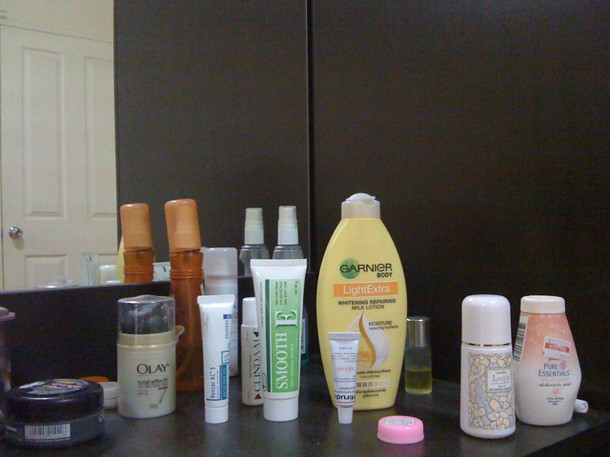The image depicts a sophisticated vanity area designed to resemble a mathematical layout. The primary feature is a black mirrored wall, creating an illusion of depth and symmetry. The reflection in the mirror reveals a white mirrored surface on the opposite side, characterized by a silver finish. This setup forms a structured arrangement of four long rectangular mirrors—two on the top and two on the bottom.

In front of the black mirror is a sleek black countertop adorned with an array of beauty products and models. The assortment includes pure essential powder and various models dusted with powder. Multiple perfume bottles add elegance to the display, accompanied by a prominent bottle of Garnier Body Express Lotion. A small tube, possibly a cosmetic or skincare item, prominently features among the collection.

Also present is "Smooth E," a type of cream known for its moisturizing properties. Among the assortment are models labeled as Thin Miasma, along with a product branded as Drake AC. An Olay product stands out on the countertop, contributing to the diverse mix of skincare items.

Additionally, there is a small round container with an unspecified product, a smaller long white tube, and a clear spray bottle situated at the back. The display also features a small white aerosol can and a round pump spray with an orange model, adorned with an orange-silver lid, completing the meticulously organized setup.